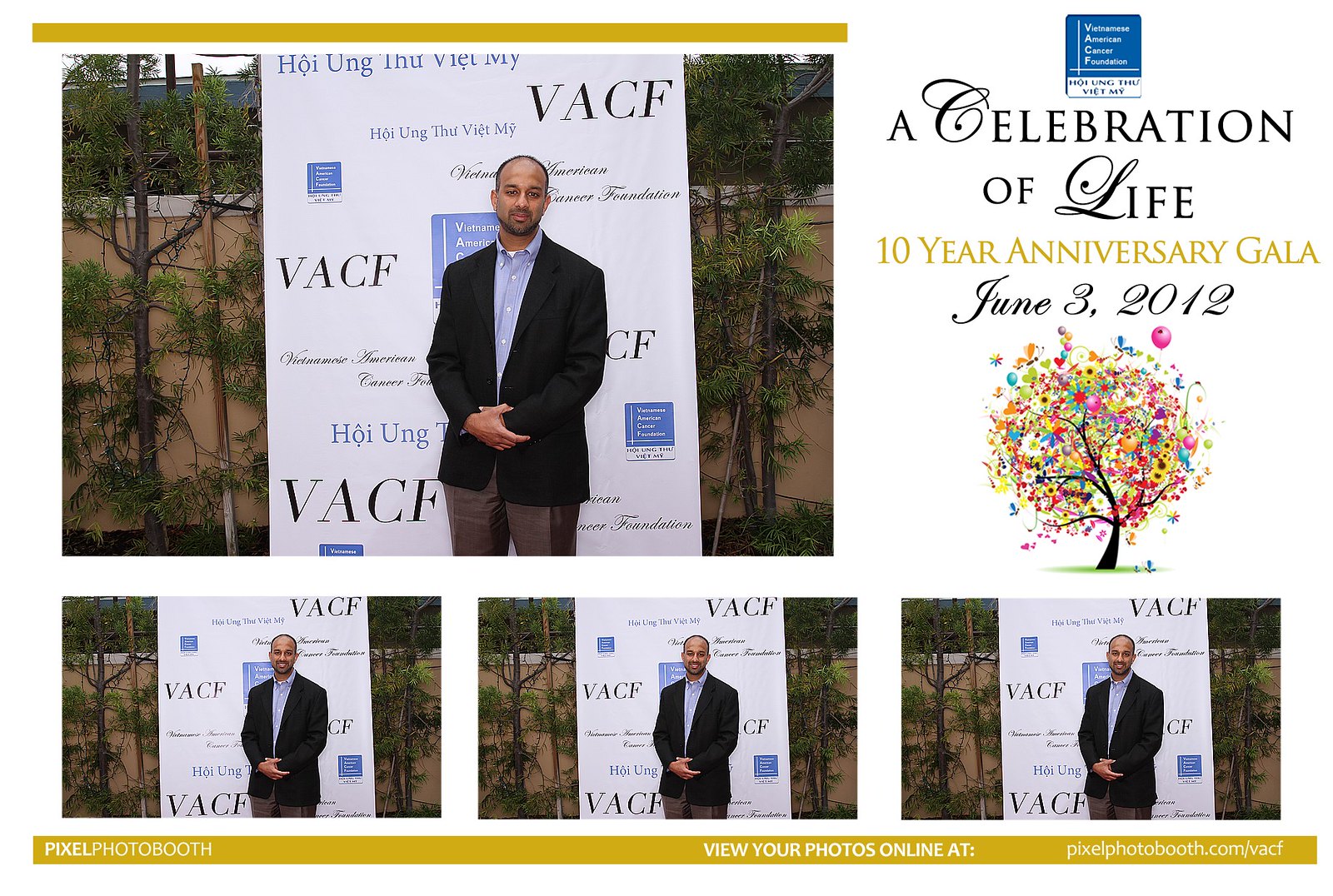The image is a rectangular card with a half-width gold border at the top and a full-width gold border at the bottom, creating a collage of several photos and text. The top left section prominently features a large photograph of an Indian man in a dark suit jacket, light blue button-up shirt, and brown pants. He stands with his hands in front of him, against a backdrop that includes a white billboard with the letters "VACF" and various symbols and writings. The background also shows a wall flanked by small trees.

To the upper right of the main photo, an emblem is displayed, along with the following text in sequence: "A Celebration of Life" in black letters, followed by "10-year Anniversary Gala" in gold letters, and "June 3rd, 2012" in black letters. Additionally, there is an illustration of a tree with multicolored leaves.

The bottom section of the card features three smaller duplicates of the primary photo, aligned above the bottom gold border, with the man exhibiting subtle smiles in these images. A text within the gold border at the bottom reads "Purcell Photography" to the left, and to the right, it states "View your photos online at" followed by a website link. The overall theme appears to commemorate the Vietnamese American Cancer Foundation's 10-year anniversary gala.